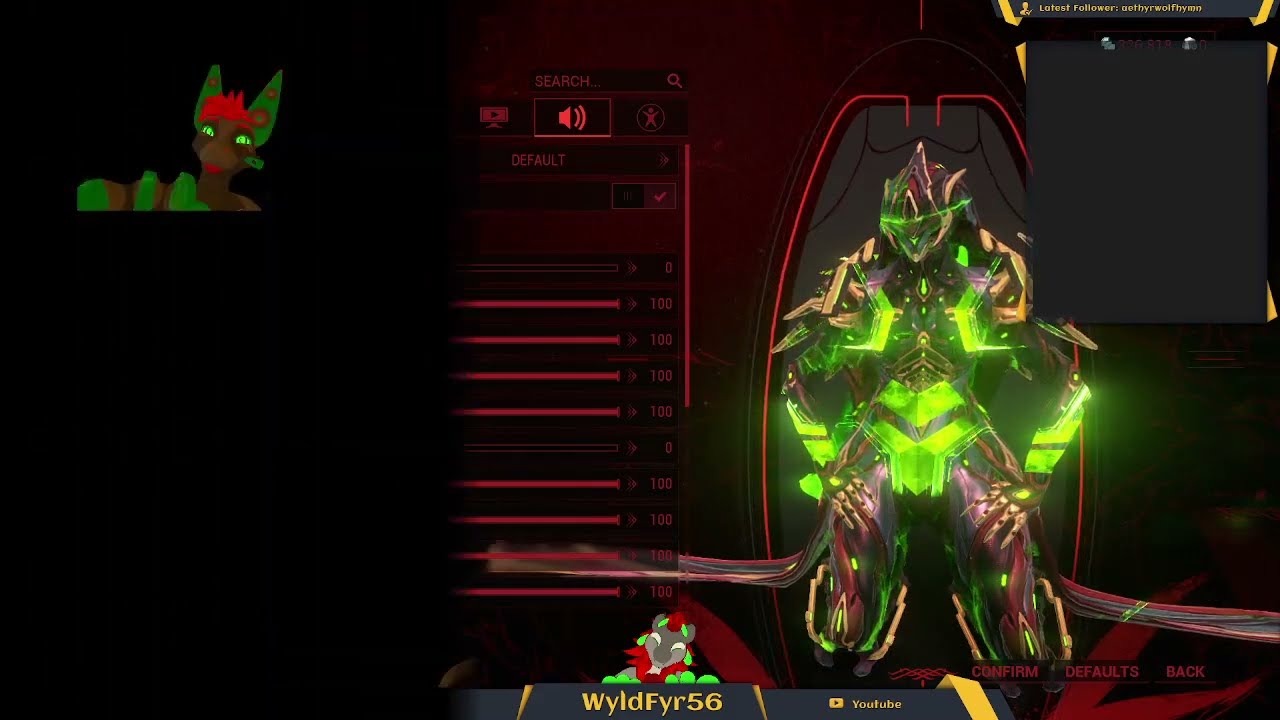In this image, a screenshot from a video game, the background is predominantly dark with sections lit up in various colors. On the right side stands a character facing the viewer, adorned in shiny green, purple, and red armor. The character has an alien face with distinguishing features like glowing green elements and pointy ears. On the left side, the screen displays some in-game stats written in red, and above these stats, in the top left corner, is a VR persona of the gamer. This avatar has brown fur, green eyes, large green bat-like ears, red hair, and green gloves, resembling an alien animal. The middle of the bottom section showcases the text "WYLDFYR56" followed by a YouTube icon and the word "YouTube." In the top right corner, there's a rectangular box with a grey background, indicating an empty chat. The overall scene suggests a character customization screen within the game, highlighted by the contrasting glowing and dark elements.